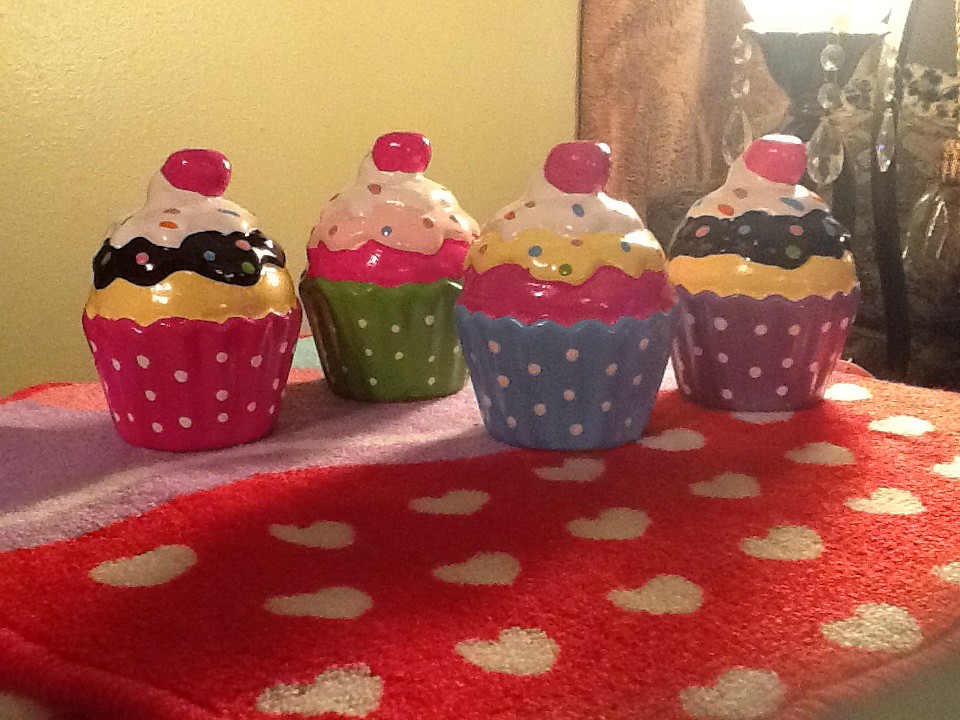This photograph is a detailed close-up of four colorful ceramic cupcakes arranged side by side on a fabric pad. The fabric pad, which appears to be a red towel with white hearts and a pink stripe, covers a surface that looks like a bathroom rug. Among the colorful layers, lines of purple and blue are also visible on the fabric. 

Each ceramic cupcake is intricately designed with a distinctive wrapper and layered frosting. The leftmost cupcake features a pink wrapper with white polka dots, topped with tiers of yellow, black, and white frosting, and finished with a red cherry on top. The second cupcake from the left has a green wrapper with white polka dots, topped with layers of hot pink, light pink, white frosting, and a red cherry. The next cupcake sports a blue wrapper with white polka dots, adorned with tiers of hot pink, yellow, white frosting, and a red cherry. The rightmost cupcake comes with a purple wrapper with white polka dots, crowned with yellow, black, white frosting, and a red cherry. 

In the background, there's a white wall with a portion of a brown curtain and a black lamp with crystal dangling accents emitting bright light.